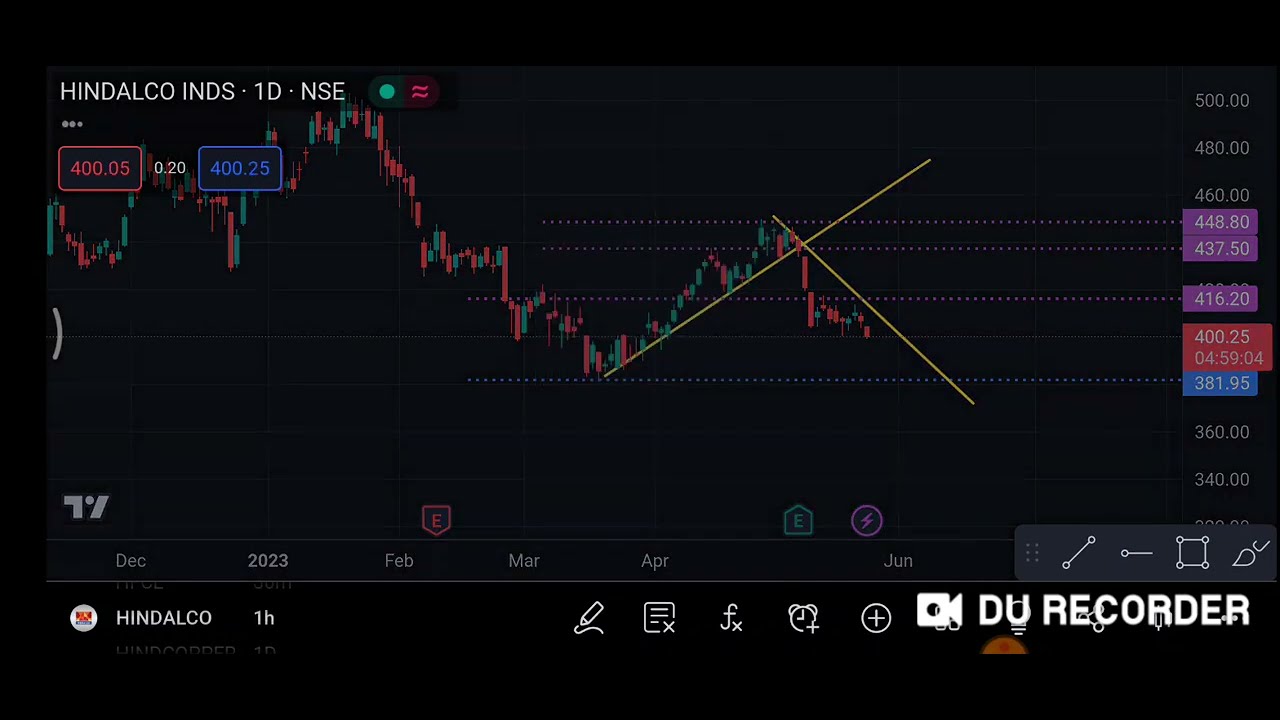The image is a rectangular screenshot with a solid black background, featuring a detailed graph in reds and greens. In the upper left-hand corner, the text "HINDALCO INDS 1D NSE" appears in white, signifying the company Hindalco Industries and a one-day timeframe from the National Stock Exchange. The graph itself shows fluctuating stock prices with prominent peaks and valleys; a significant rise is followed by a sharp decline, and then it briefly climbs again. Yellow lines indicate key movements. On both the left and right vertical axes, numerical data is displayed. The bottom section of the graph includes a timeline with labels for December 2023, February, March, April, and June, though it's unclear if these are past dates or future projections. In the lower left-hand corner, additional text reiterates "HINDALCO 1H" suggesting a one-hour glimpse. Also, overlaid text and a logo next to a video camera icon, labeled as "DU Recorder" or "DV Recorder," indicate that this image was captured using a screen recording tool.